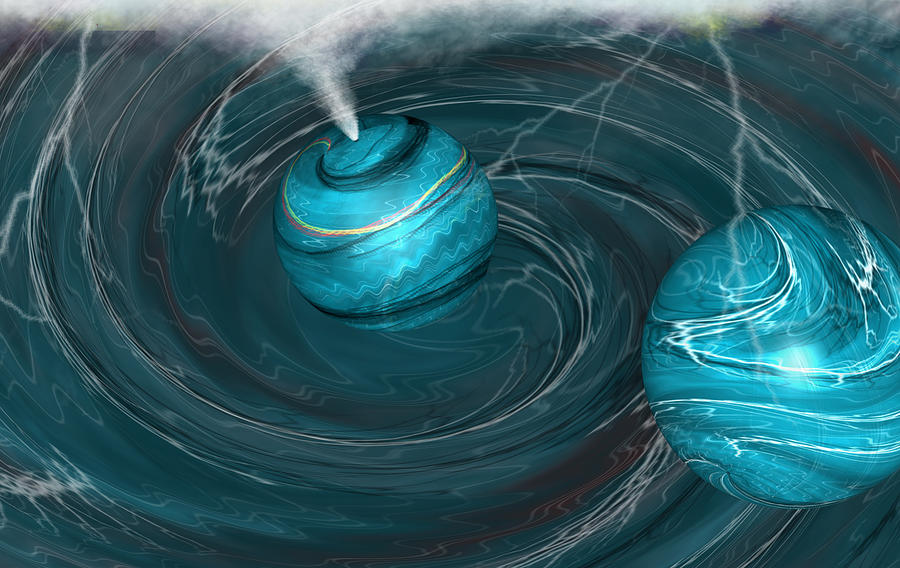In this digital art image, we see two blue planets being pulled into the swirling, spiral formation of a massive whirlpool or tornado. The whirlpool, resembling a hurricane or possibly even the opening of a black hole, is predominantly blue with hints of green, brown, and white. One planet is centrally located within this dynamic spiral, while the other is positioned towards the right, on the outskirts of the vortex. From the center planet, white steam or smoke emanates, spreading around it. Additionally, there are lightning jolts visible in the background, contributing to the dramatic and otherworldly atmosphere of the scene. The overall image has been meticulously crafted with computer-generated imagery (CGI), showcasing the detailed and immersive nature of digital art.